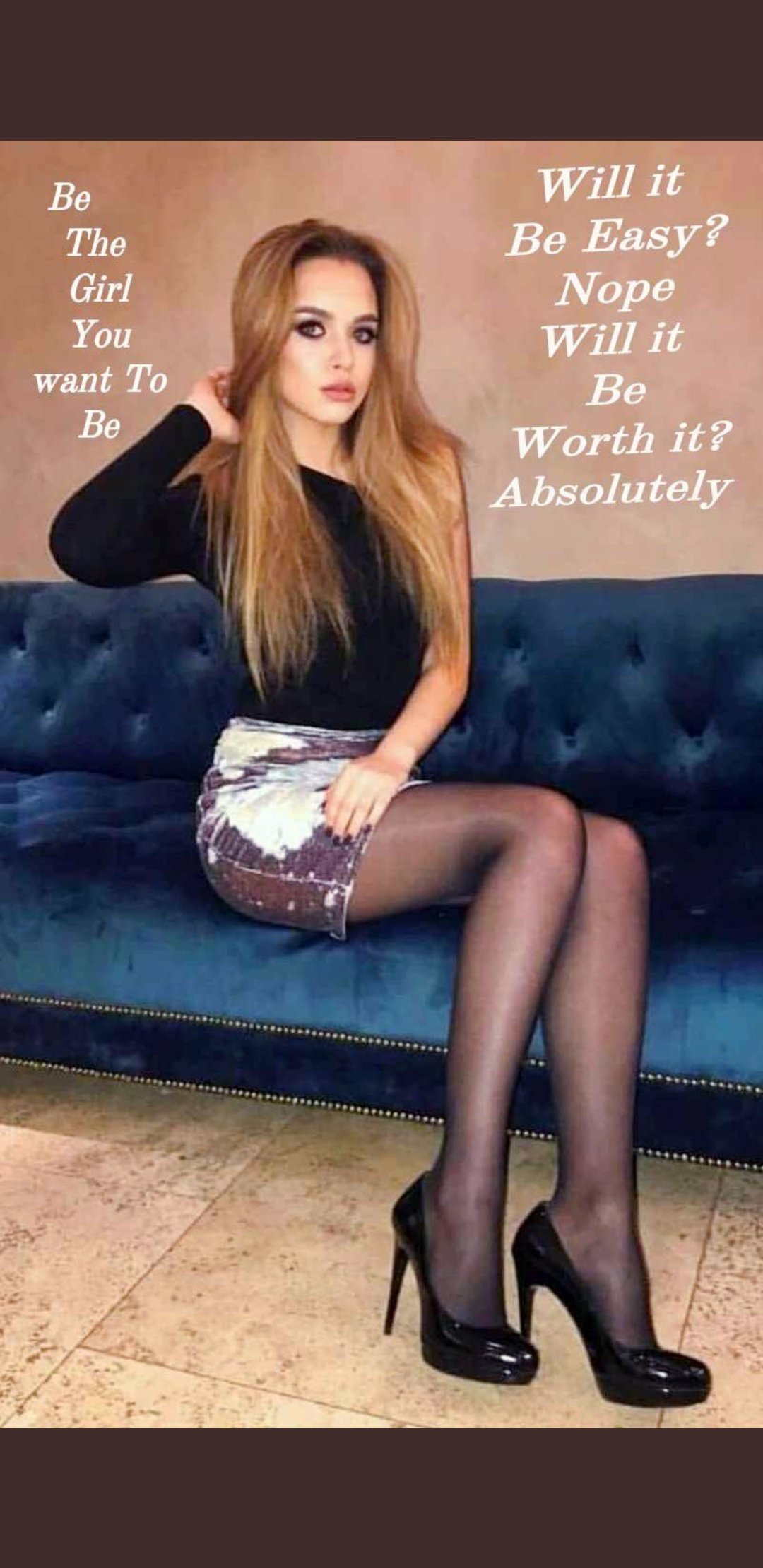The image is a vertically-oriented photograph framed by thick brown borders at the top and bottom. In the center, a young woman with long, light brown hair cascading in front of her chest sits on a blue, tufted velvet sofa adorned with brass tacks. She is posed slightly turned to the right, facing forward. Her right arm is bent with her hand placed behind her head, while her left arm rests on her lap. She wears an asymmetrical, off-the-shoulder black top with one sleeve, along with a silver sequined miniskirt. She completes her outfit with sheer black stockings and black high heels, her feet touching the cream-speckled porcelain tile floor below. Behind her, there is white text on the wall reading, "Be the girl you want to be" on the left and "Will it be easy? Nope. Will it be worth it? Absolutely" on the right. The image is brightly lit, showcasing the woman clearly, with no other people present.